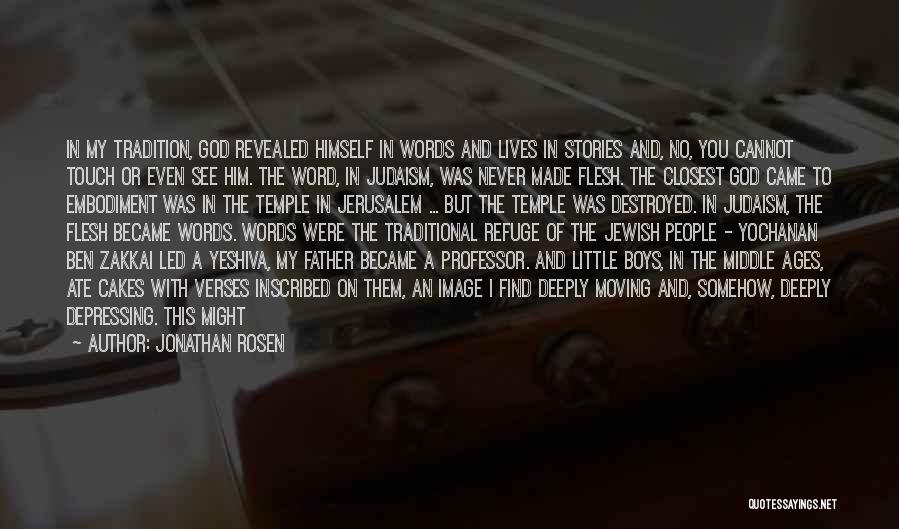The image is a horizontally oriented photograph with a dim, blurry background that resembles a view of guitar strings stretching to the left. Superimposed over this backdrop is a substantial quote, rendered in white text, which reads: "In my tradition, God revealed himself in words and lives in stories. And no, you cannot touch or even see Him. The word in Judaism was never made flesh. The closest God came to embodiment was in the Temple in Jerusalem. But the Temple was destroyed. In Judaism, the flesh became words. Words were the traditional refuge of the Jewish people. Yochanan ben Zekai led a yeshiva. My father became a professor and little boys in the Middle Ages ate cakes with verses inscribed on them, an image I find deeply moving and somehow deeply depressing. This might." The quote is attributed to the author Jonathan Rosen, with the source "quotes sayings dot net" noted in the bottom right corner. The image's background colors are subdued, featuring tones of grey, brown, black, beige, and white. The overall style suggests an internet meme designed to convey a reflective and somber message about the enduring power of words in Jewish tradition.